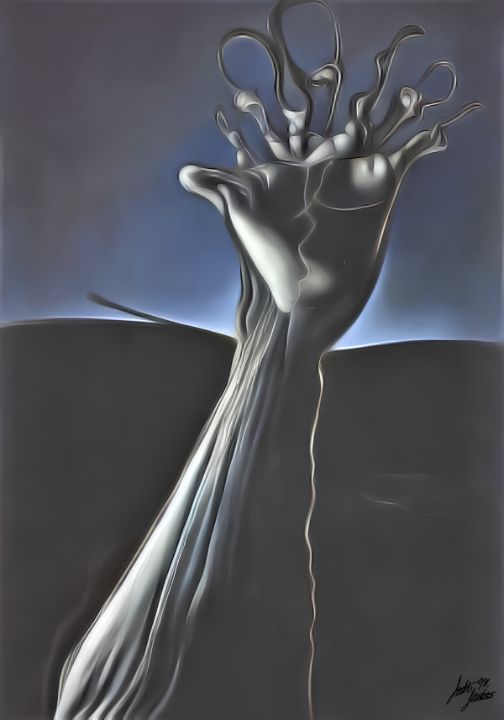This detailed portrait layout image features a surreal and eerie setting with a predominant blue-gray upper half transitioning into a black lower half background. Emerging from the bottom center of the frame is a warped, disfigured forearm and hand that appears to be morphing. Instead of typical fingers, the appendages transform into various tools such as a dental pick, a hook, and scissor handles, giving the impression of a melting metamorphosis. The hand itself is rendered in different shades of grays, blacks, and whites, adding to the unsettling atmosphere. In the lower right corner, there is an illegible black cursive autograph, likely from the artist. The entire composition is dark and haunting, with no other colors, text, or people, set against a backdrop that transitions from a dark gray resembling a mountain up to a smoky, hazy blue-gray sky.